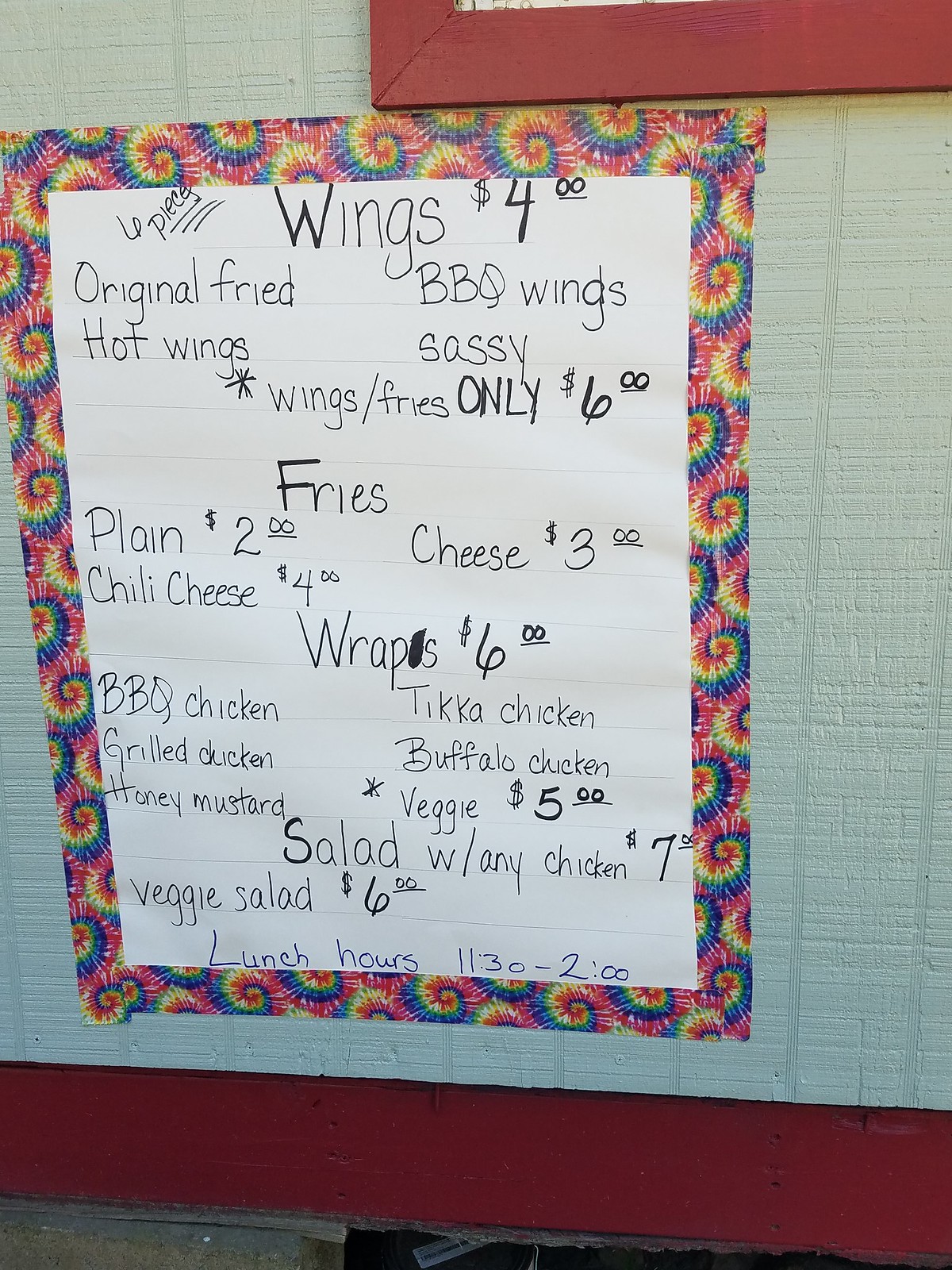The image showcases a vivid scene featuring a red-colored wall, mostly covered by a white plaster wall, with approximately 90% of the red surface hidden. At the bottom of the image, a strip of the red wall is visible. Topping the scene, there is a partial view of a red wooden frame.

Within the frame, a poster is mounted on the white plaster wall. The poster features rainbow-colored spiral edges with a pink background border. The content of the poster is primarily a restaurant menu printed on white paper. 

At the top of the menu, it lists:
- Wings: $4 for a 6-piece order.

The menu then details various types of wings:
- Original Fried (left side)
- Barbecue Wings (right side)
- Hot Wings (left side)
- Sassy Wings (right side)

Additionally, it mentions:
- Wings and Fries combination: $6
- Fries: $2 for plain, $3 for cheese, and chili cheese options on the right.

Further down, the menu lists:
- Wraps: $6, with different flavors available.
- Salads with any chicken: $7
- Veggie Salad: $6

Lastly, the menu indicates the lunch hours, which are from 11:30 AM to 2 PM.